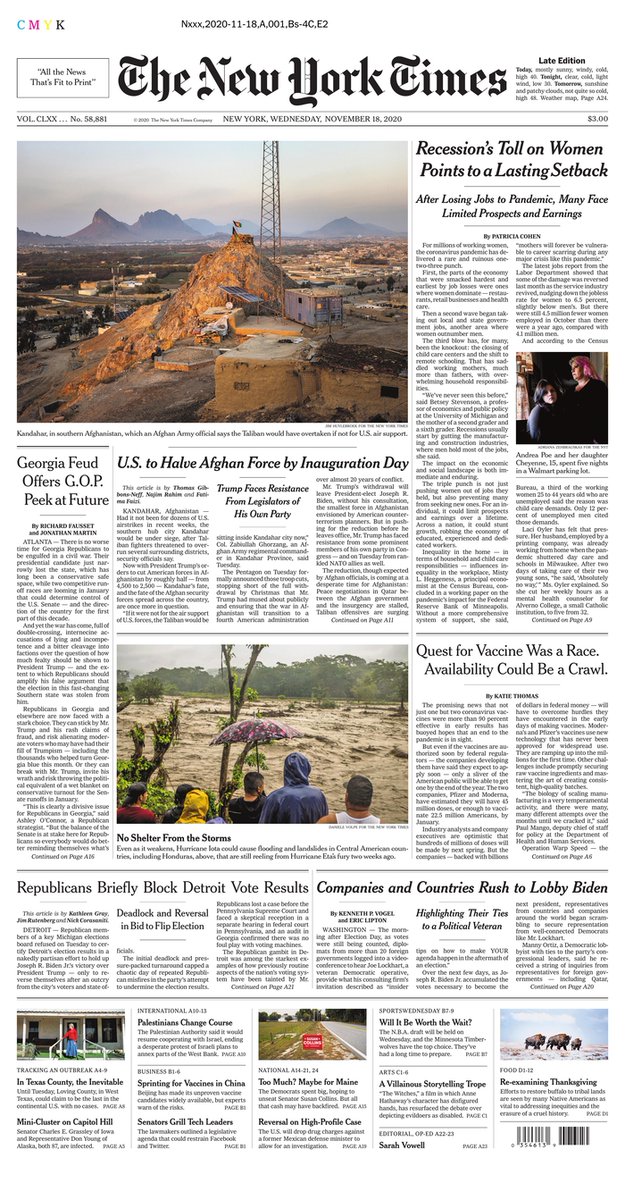This is a detailed screenshot of a digital edition of The New York Times. Positioned at the top left of the title is a small box featuring the newspaper's motto, "All the News That's Fit to Print." On the top right, it indicates that this is the "Late Edition." Directly beneath the masthead, a thin border signifies the newspaper's date and location: "New York, Wednesday, November 18, 2020."

The main headline reads, "U.S. to Help Afghan Force by Inauguration Day," accompanied by a panoramic photo of a town in Afghanistan. Prominently placed on the right side is an article titled "The Recession Toll on Women Points to a Lasting Setback" by Patricia Cohen, including an image of two women.

Another significant article, "Quest for Vaccine Was Erased; Availability Could Be a Crawl," is situated in the center-right of the page. A striking photo under this headline captures people observing floodwaters, with the caption "No Shelter From the Storm."

Additional articles feature headlines like "Republicans Briefly Blocked Detroit Vote Results" and "Companies and Countries Rushed to Lobby Biden." At the bottom right corner of the page, a barcode is visibly printed.